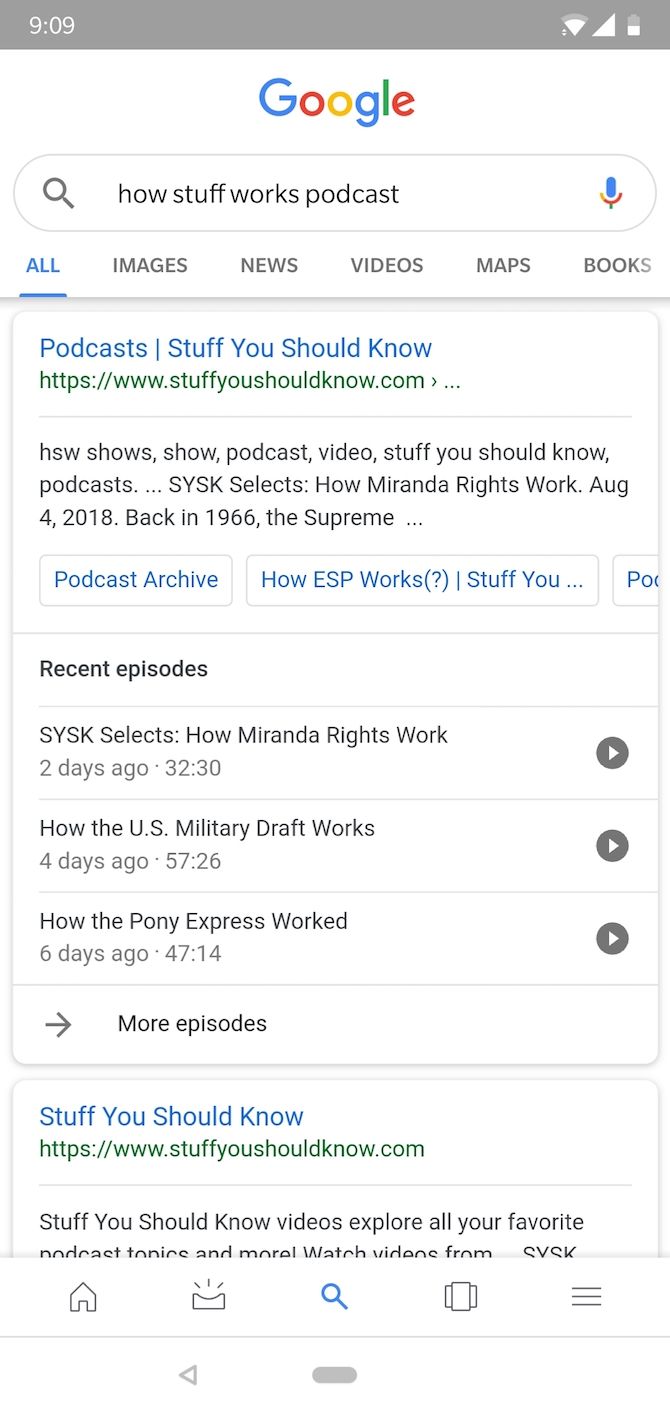This screen capture depicts a Google search result for "How Stuff Works podcast" on a smartphone. At the top, a gray bar displays the time "9:09" along with a white Wi-Fi icon and a battery icon. Below, the Google logo in its signature blue, red, yellow, and green colors is visible above the search box which contains a magnifying glass icon. The search query "how stuff works podcast" is entered in the box. A microphone icon in blue, red, and green is situated to the right of the search bar.

Underneath, there are submenus with options: "All" in blue, followed by "Images," "News," "Videos," "Maps," and "Books" in gray. The first search result features a blue hyperlink "Podcast Stuff You Should Know" followed by a green clickable website address. A gray text snippet "hsw shows show podcast video Stuff You Should Know Podcast sysk selects How Miranda Rights Work Aug 2018 Back in 1966, the Supreme..." is shown but cuts off mid-sentence.

Further down, boxed sections in white with blue text showcase available podcast archives. Each entry lists a title, a timestamp, and a small play button. The first few entries are: "SYSK Selects: How Miranda Rights Work" (2 days ago, 32 minutes 30 seconds), "How the US Military Draft Works" (4 days ago, 57 minutes 26 seconds), and "How the Pony Express Worked" (6 days ago, 47 minutes 14 seconds). A gray arrow labeled "More episodes" promises additional content.

Another search result headline in blue "Stuff You Should Know" with a green website address is shown, above a truncated gray blurb that reads "Stuff You Should Know videos explore all your favorite podcast topics and more. Watch videos from SYSK..."

At the bottom of the screen, a white menu bar displays several icons in gray: a house icon, a box with squiggly lines, a piece of paper with lines, and a back arrow in a gray bar. The magnifying glass icon is highlighted in blue, indicating the active search function.